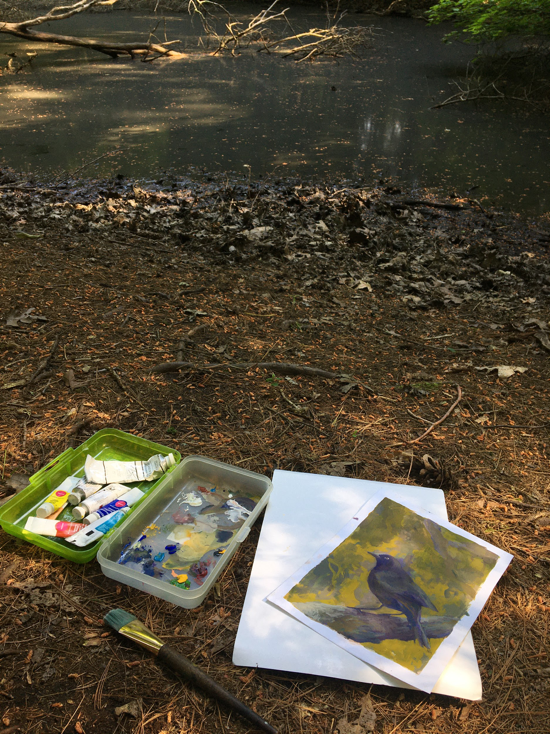In this photograph, we observe an artist's workspace, suggesting an attempt at creating a painting. In the foreground, there is a white drawing pad featuring a dark-colored bird sketched against a blended yellow and bluish background. Nearby lies a paintbrush, its bristles stained with blue paint. The brush has a gold ferrule and a brown handle. To the immediate left of the white pad, there is a clear plastic palette containing small pools of various paints. Adjacent to this is a green plastic palette holding a diverse array of paint colors.

Moving to the background of the photograph, the scene shifts to an outdoor setting featuring a small pond. A fallen tree partially submerged in the murky, dark water adds a natural, rustic element to the composition. Surrounding the pond is a mix of dark, weathered ground with orange and black hues from the lighting and surrounding vegetation. The overall scene combines elements of artistic creation with the raw beauty of nature, capturing a moment of tranquil creativity.